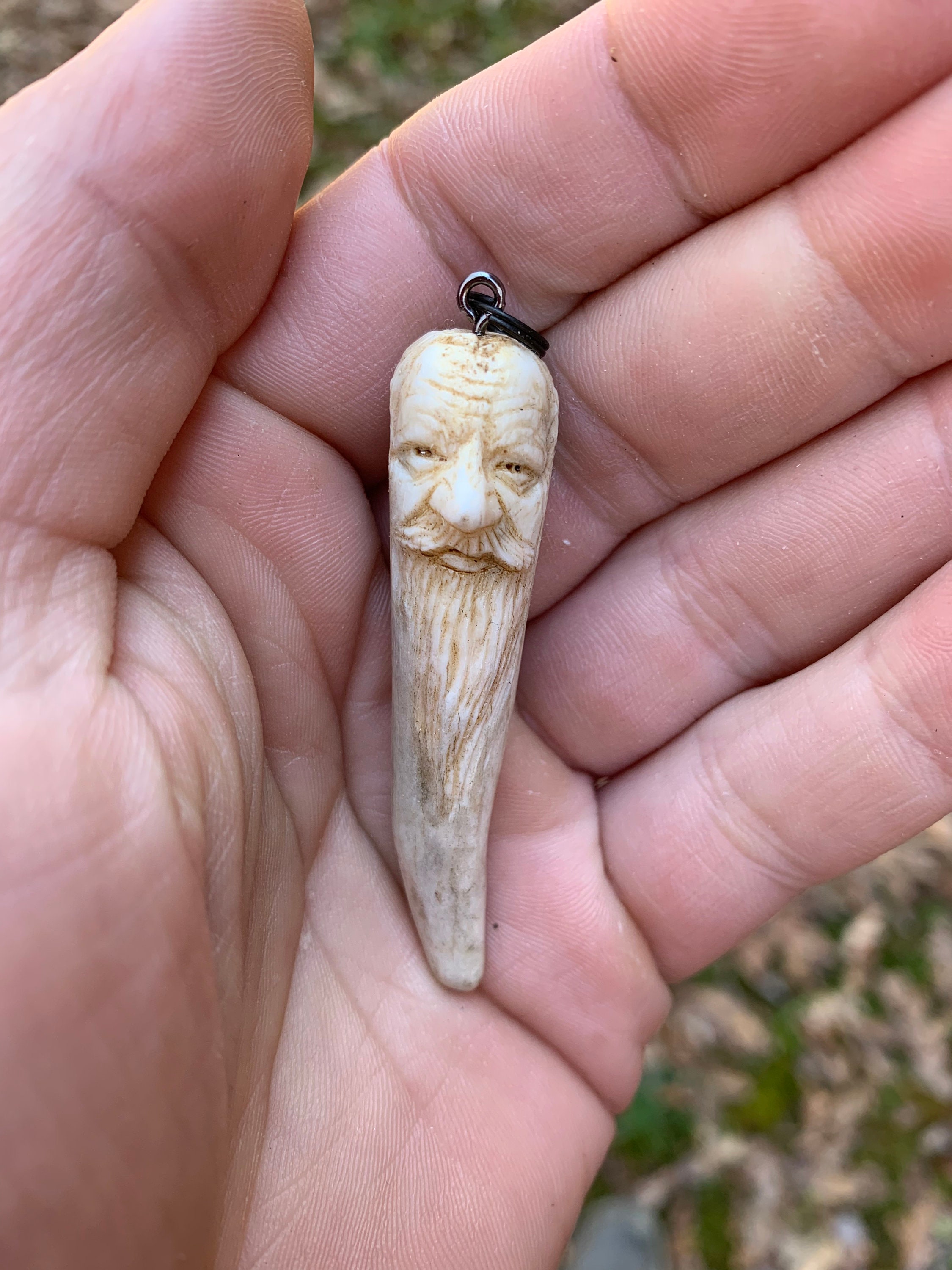In this vertical, close-up photograph, a left hand is prominently displayed, emerging from the lower left corner. The hand is positioned palm up, revealing the thumb and three-quarters of each finger against a backdrop of intricate palm lines. In the center of the hand's palm rests a meticulously carved ivory pendant, shaped reminiscent of a tooth. The pendant features a lifelike human face with striking details: a wrinkled forehead, a bulbous nose, aged eyes, and a flowing beard and mustache that extend from the pendant's center down to its narrowing tip. The level of detail in this close-up allows for the observation of both the fine craftsmanship of the pendant and the aged characteristics of the hand, suggesting it belongs to an older individual.